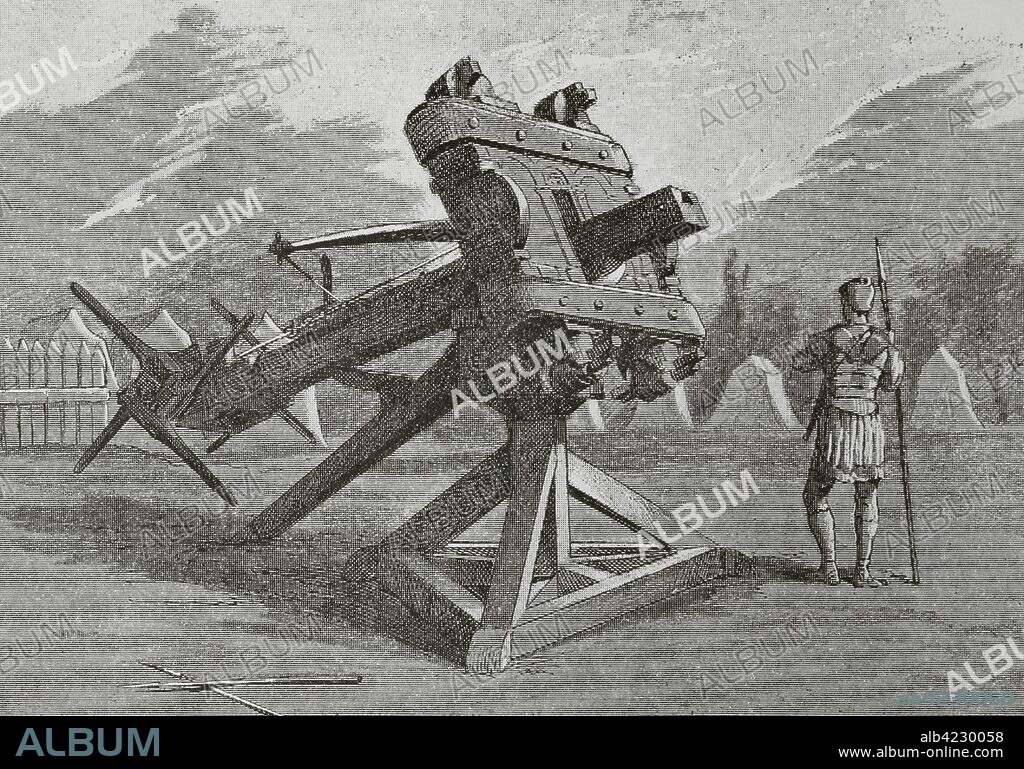This black and white image appears to be a vintage, computer-generated or pencil-drawn illustration depicting a medieval scene. Dominating the scene is a large, wooden siege machine, likely a ballista, characterized by its crossbow-like structure and a winch mechanism at the back. Adjacent to this formidable weapon stands a warrior outfitted in detailed armor, including a metal helmet and an armored torso. He wields a long spear in his right hand and wears a pleated skirt and flat boots. The warrior seems to be in a grassy area, surrounded by dirt, with subtle background elements like hills, a wooden fence, and outlines of tents suggesting a encampment site. The entire illustration is overlaid with the word "album" repeatedly in white, creating a watermark effect, and at the bottom, there is a black border containing the text "album" in blue alongside the website www.albumonline.com.